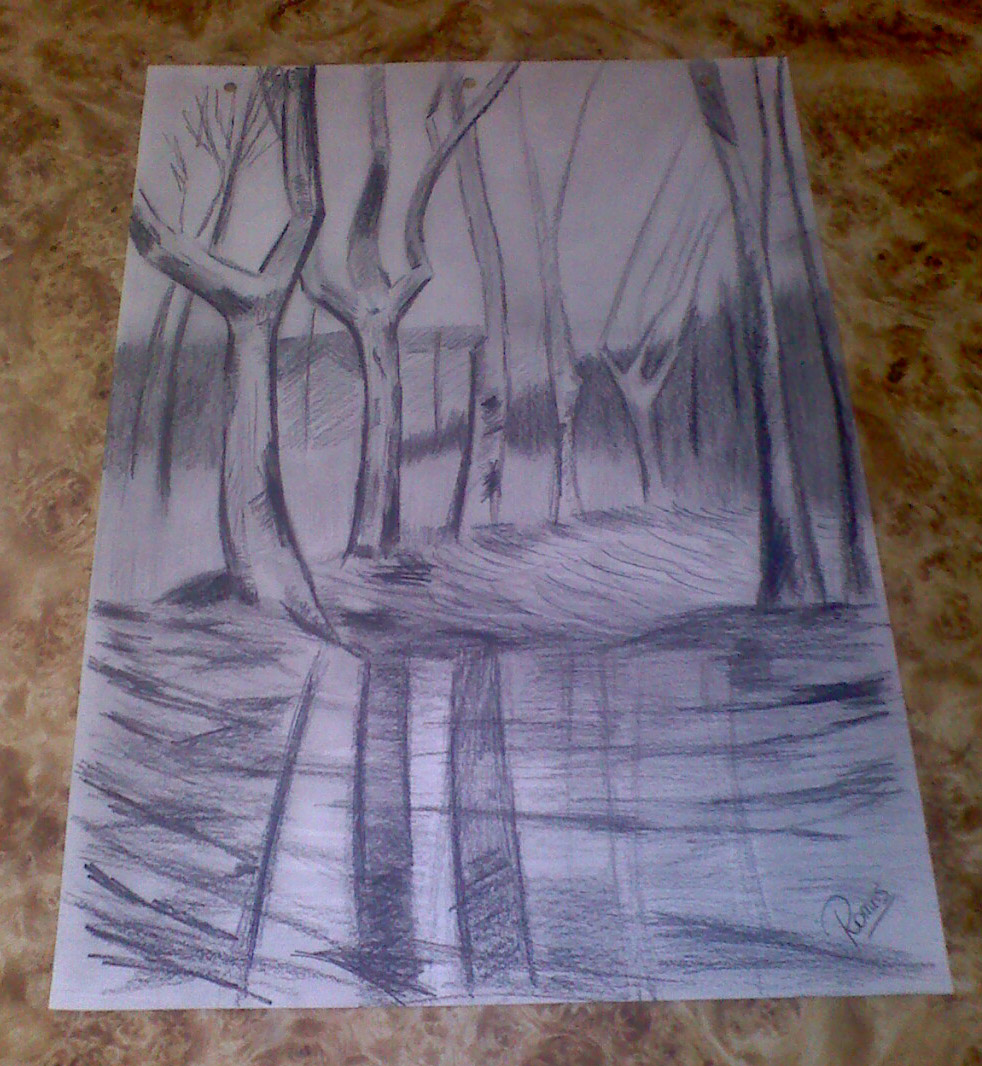The photograph captures a compelling graphite pencil drawing on a white canvas, featuring a hauntingly desolate forest scene. The central pathway or roadway leads the viewer's eye through an array of barren trees, stark and leafless, aligning the sides of the path. Intricately sketched, the trees stand prominent against a backdrop of negative space, lending an air of desolation and somber beauty to the artwork. In the distance, a densely packed forest looms, merging into the background beneath a light gray, overcast sky that enhances the melancholic atmosphere of the piece. The artist's signature is elegantly placed at the bottom right corner, completing the composition. The canvas itself rests on a light tan granite countertop, providing a warm contrast to the cool tones of the drawing.